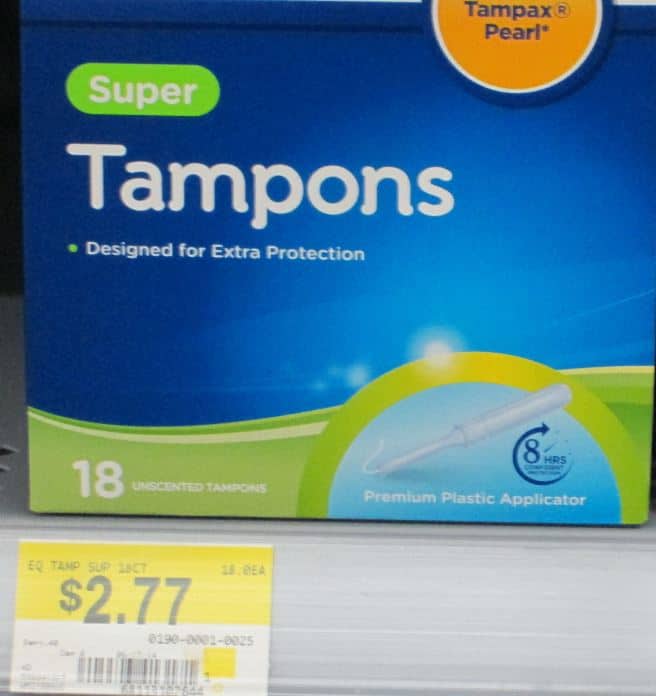This square-shaped photograph, taken indoors at a store, displays a close-up of a product on a metal shelf. The featured item is a blue and green box of tampons with distinctive design elements and text. Prominently, a circular orange area at the top right reads "Tampax Pearl." Below that, enclosed in a green rounded rectangle, the word "super" appears in white letters. The center of the box displays the text "tampons" in white against the blue background, followed by "designed for extra protection." Toward the bottom, the green area curves decoratively, stating "18 unscented tampons" alongside an image of a tampon and the label "premium plastic applicator." An additional logo indicates "8 hours" of protection. The box rests on a gray metal shelf, and in the lower left corner of the image, a yellow and white price tag reads "EQ TAMP SUP 18" with a barcode and price of $2.77.